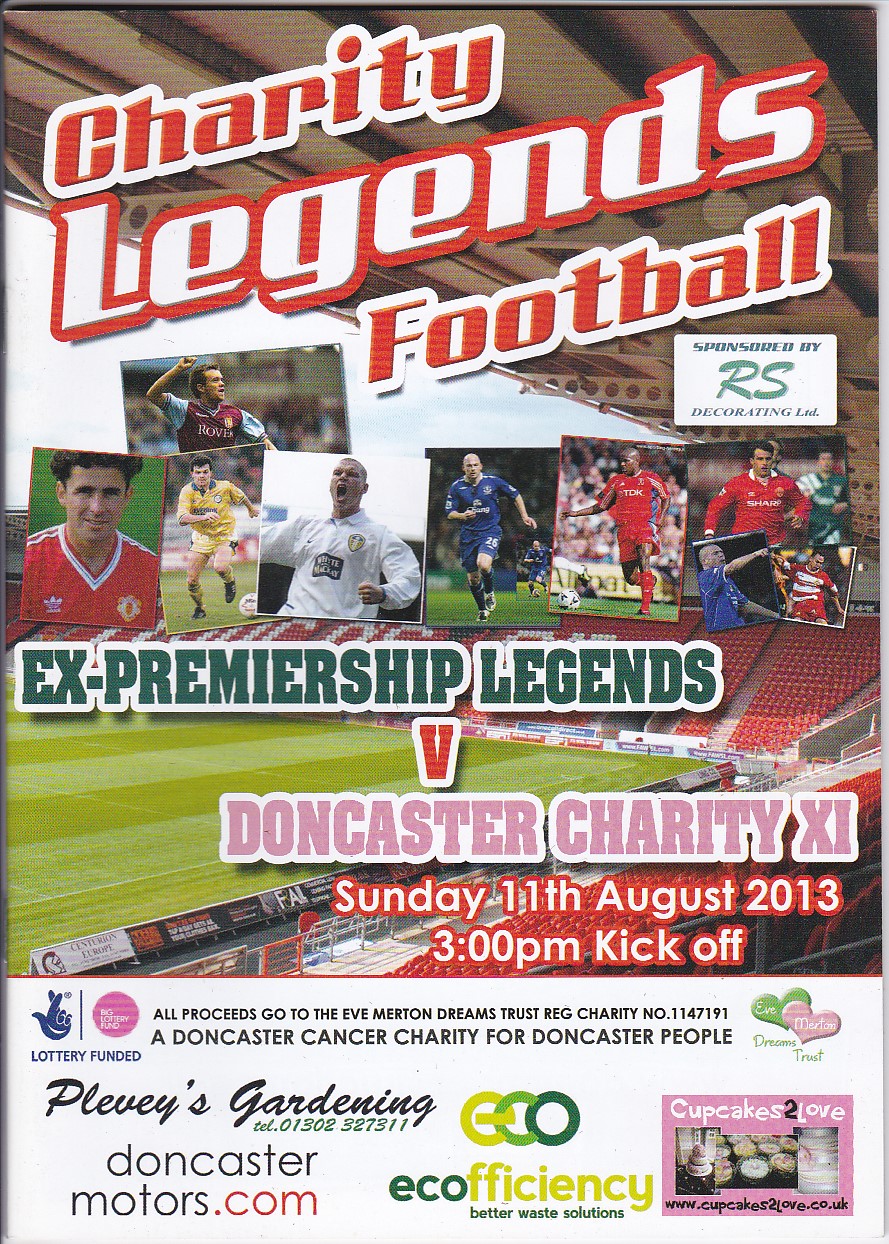The image appears to be the cover of a game day program or magazine for an event titled "Charity Legends Football." The title is prominently displayed at the top in large diagonal text with "Charity" in red letters outlined in white, "Legends" in white letters outlined in red, and "Football" in red letters outlined in white. Below the title, there's a small square on the right side that states "Sponsored by RS Decorating Limited." 

Across the center of the cover, there's a row of small square pictures featuring various soccer players in different uniforms. Beneath these images, the event details are written in green letters outlined in white: "X-Premiership Legends v. Doncaster Charity XI." The date and time are clearly marked as "Sunday, 11 August 2013, 3pm kickoff," with the font being white outlined in red.

Towards the bottom, a solid white rectangular banner spans the width of the page, listing the sponsors and additional details. In black font, it indicates that "All proceeds go to the Eve Merton Dreams Trust, Reg Charity number 1147191, a Doncaster Cancer Charity for Doncaster people." The banner also features logos and names of various sponsors including Plevy's Gardening, EcoEfficiency, and DoncasterMotors.com. The background of the entire cover appears to be a photo taken from the stadium seating, showing a view of the field under the overhang, adding a dynamic contextual backdrop to the information provided.